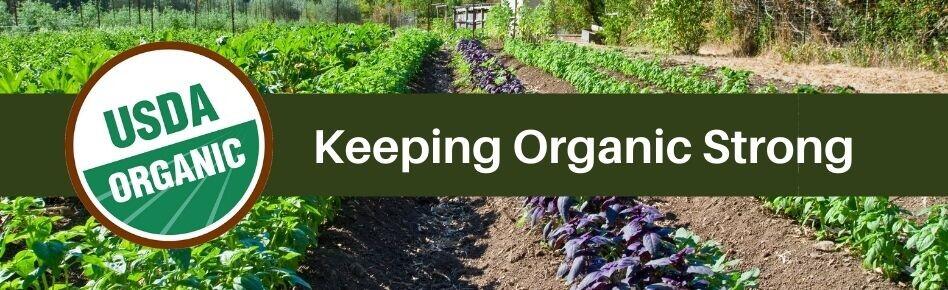The horizontal banner photograph features rows of meticulously cultivated vegetables growing in a farm field, with patches of sandy brown dirt between them. The farm is vibrant with green leaves, green plants, and a row of intriguing purple-colored plants, possibly purple lettuce. In the background, the farmland is marked by ridges and bordered by bushes on the right side. Dominating the upper portion of the image is a horizontal olive green bar spanning about one-third of the photograph's width. This bar contains a bold white text that reads, "Keeping Organic Strong." On the left side of the bar, there is a circular logo with a deep maroon red outline. Inside the circle, the top half is white with the green text "USDA," while the bottom half is green with diagonal white lines resembling crop rows, featuring the white text "ORGANIC."